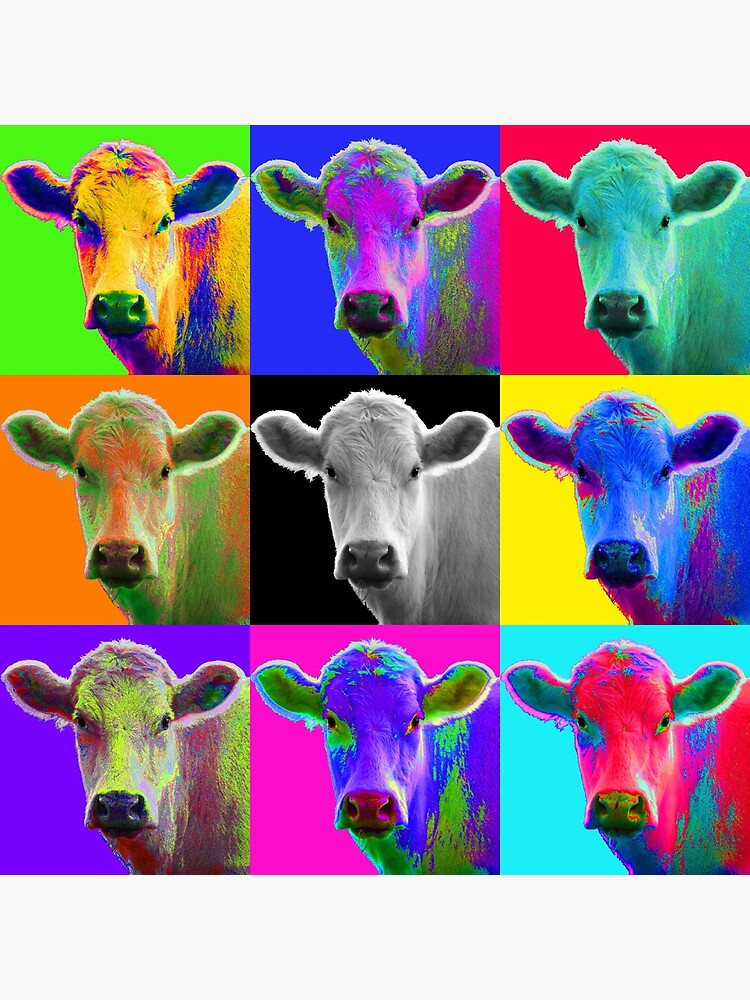The image is a vibrant, multi-colored artistic print composed of nine individual square photographs of the same cow's head, each rendered in different color schemes similar to an Andy Warhol-esque pop art style. The cow's eyes are consistently black in all images. The background and cow colors vary significantly, creating a neon and unrealistic visual effect. 

- **Top Row (left to right):**
  1. Cow: Bright orange, Background: Neon green
  2. Cow: Dark green with neon purple highlights, Background: Dark blue
  3. Cow: Pale neon green, Background: Bright red

- **Middle Row (left to right):**
  1. Cow: Dark and light green with orange tinges, Background: Orange
  2. Cow: Black and white (central photograph)
  3. Cow: Purple-blue with red highlights, Background: Bright yellow

- **Bottom Row (left to right):**
  1. Cow: Light green and red pastel, Background: Purple
  2. Cow: Dark purple with neon green markings, Background: Bright pink
  3. Cow: Bright red with green around the eyes and snout, Background: Light blue

The overall layout lacks a definitive border or set background and is characterized by its use of strikingly vibrant and neon colors, enhancing the visual impact of the repeated cow's head looking directly at the camera.